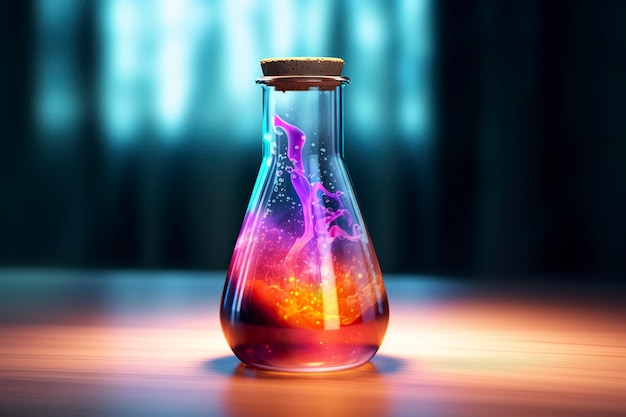This image features a pear-shaped glass bottle, sealed with a cork, sitting on a wooden table. The table, illuminated by a circle of light, reflects the vibrant colors within the bottle. Inside, a mesmerizing mixture of colored oils and liquid creates a lava lamp-like effect. The colors, including vivid pink, violet, lavender, coral, brown, yellow, and a hint of black, swirl and blend, forming suspended shapes that transition from red and orange at the bottom to purple toward the top. Blue splatters can be seen inside the bottle, extending from the liquid up to the neck. The background is blurred, predominantly black with shades of teal blue that suggest a window, obscured by shadows. The overall scene is bathed in a mysterious glow, highlighting the surreal beauty of the colorful liquid in the bottle.